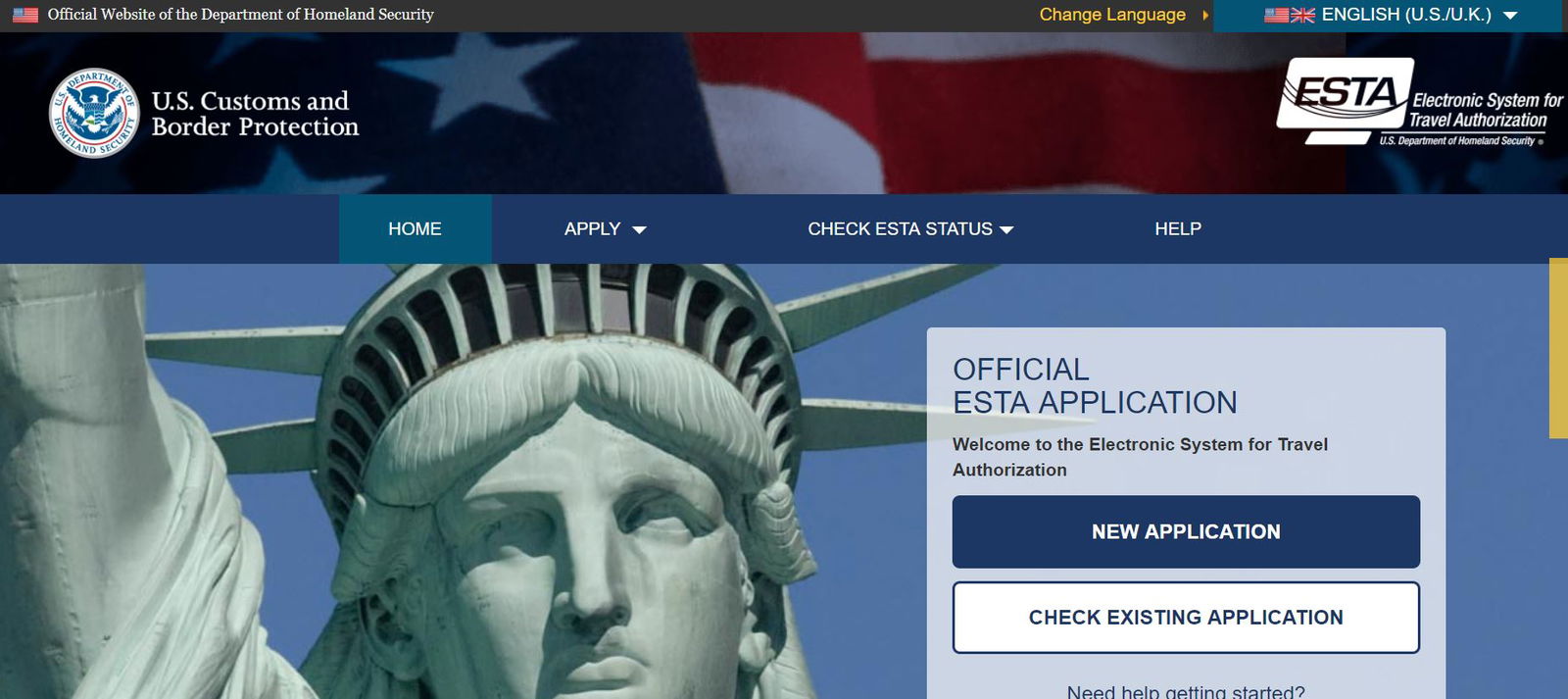Homepage of the U.S. Customs and Bureau of Protection's Togami Website

The homepage of the Togami website, dedicated to the U.S. Customs and Bureau of Protection, presents a formal and organized layout aimed at assisting users with the Electronic System for Travel Authorization (ESTA). 

**Top Section:**
- **Logo and Title:** On the top left, the organization's logo is prominent, with white text reading "U.S. Customs and Bureau of Protection."
- **Electronic System for Travel Authorization:** To the right of the logo, the title "Electronic System for Travel Authorization" is displayed.
- **Language Selection:** Towards the right edge at the top, there is a symbol indicating language choice, followed by the text "Choose Language." The current selection shows "English (U.S.-U.K.)."

**Header Border:**
- An American flag subtly serves as the background of the header.
- Below the header is a navigation bar featuring three primary options: "Home," "Apply," and "Check ESTA Status."

**Main Content:**
- **Visual Element:** The main body of the homepage features an impressive image of the Statue of Liberty, focusing on its head and raised arm against a backdrop of the sky.
- **Welcome Message:** To the right of this image, the text reads "Official ESTA Application" and "Welcome to the Electronic System for Travel Authorization."
- **Action Buttons:** A prominently displayed blue hyperlink box labeled "New Application" invites users to start the process. Below this button, another option in white text reads "Check ESTA Application," enabling users to check their application status.

**Departmental Note:**
- To the left of the entire page, a note indicates that the site is the "official website of the Department of Homeland Security."

These details collectively offer a comprehensive look at the primary elements and navigation options available on the U.S. Customs and Bureau of Protection's Togami website homepage, ensuring users can efficiently access ESTA-related services.